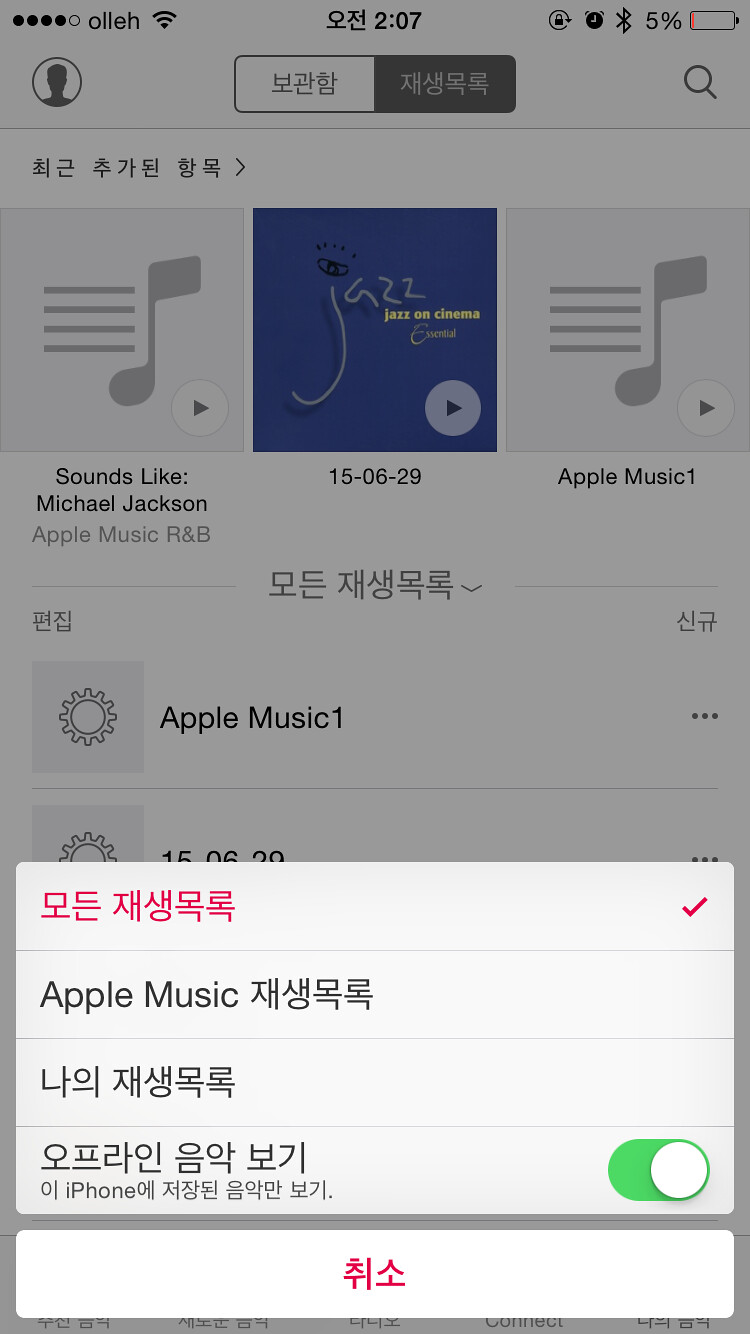The image depicts a smartphone screen predominantly featuring Japanese text with some English elements. In the upper left corner, the symbols "O-L-L-E-H" are visible beside a Wi-Fi icon comprising five circles, four of which are filled. The time reads "207" following a Japanese character, and the device power is at 5%. The central part of the screen lists music tracks, including "Jazz on Cinema," dated "150629," alongside start buttons marked by musical notes. "Sounds Like Michael Jackson, Apple Music R&B" is also displayed prominently. To the right, "Apple Music One" is mentioned multiple times. A gear icon and a trio of dots appear further down, indicating settings and additional options. At the bottom, the word "iPhone" is visible in English along with a green toggle switch and additional Japanese characters. The screen is dimmed slightly due to a red-checked pop-up notification displaying unreadable symbols and a red checkmark to the right.